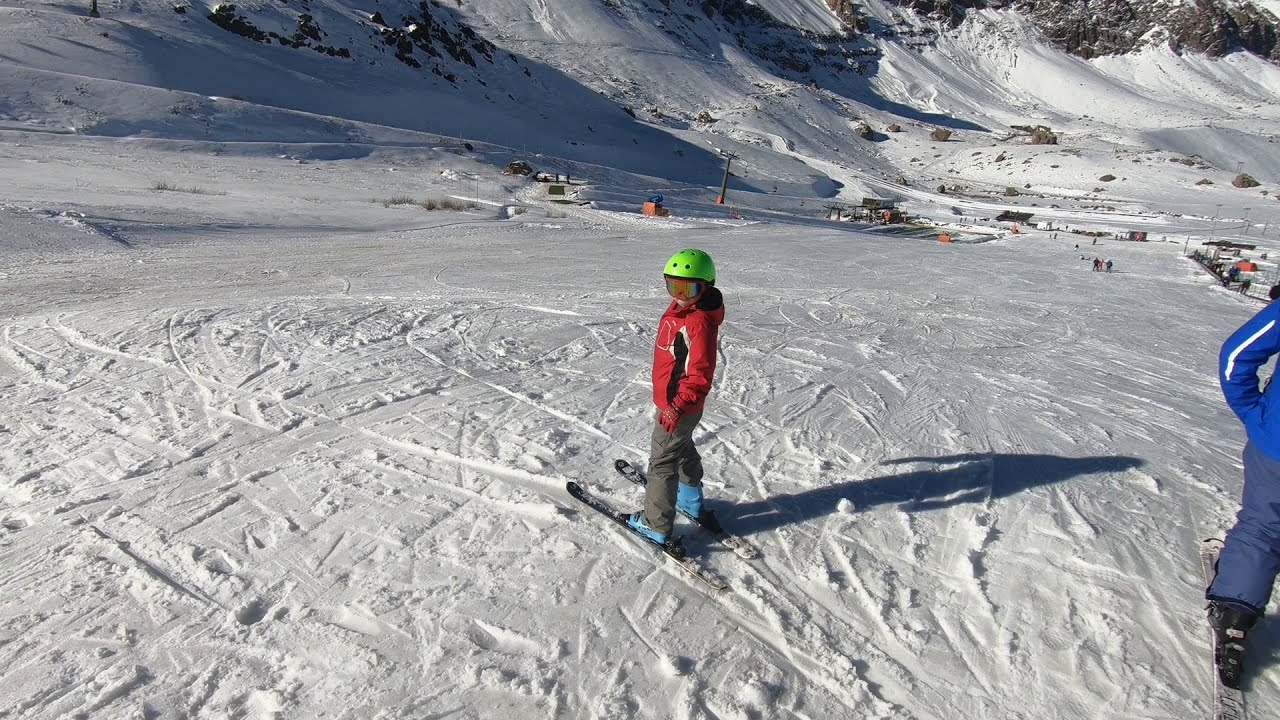In this horizontally rectangular, full-color photograph taken outdoors on a winter's day, the scene captures a ski resort from the perspective of a ski slope near its top. The foreground prominently features a small child dressed in a red jacket, blue boots, dark gray snow pants, red gloves, a yellow helmet with a visor, and ski goggles. The child stands on skis, poised to descend the hill. To the right, part of an adult figure can be seen wearing a blue jacket, light bluish-gray pants, and black ski boots; they are also on skis but neither skier holds ski poles.

Behind them, the snow-covered hill is marked with numerous tracks from other skiers, indicating heavy usage. In the middle and lower portions of the image, scattered further down the hill, are several skiers alongside structures that suggest ski lift stations, characterized by small buildings and towers. The jagged, rocky upper portion of the slope signals a hazardous area not suitable for skiing. The photograph captures the late evening sun casting long shadows, adding to the tranquil yet dynamic atmosphere of the ski slope and the distant ski resort town below. The sky itself is not visible in the image.